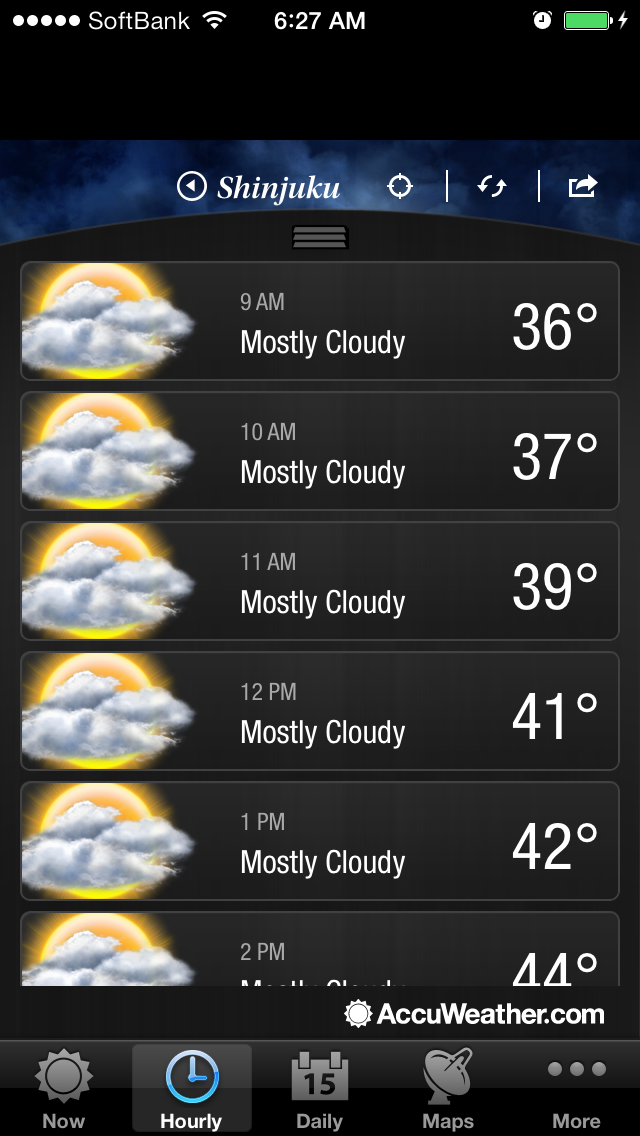**Detailed Caption:**

This image is a screenshot of an hourly weather forecast displayed on the AccuWeather mobile app. At the top of the screen, there are five horizontal white dots on the upper left, followed by the text "SoftBank." A Wi-Fi icon indicates two bars of signal strength. The time, centered at the top, reads 6:27 AM. Adjacent to it is an alarm clock icon, showing that an alarm is set. The nearly full battery icon is green with a lightning bolt, indicating it is charging.

Underneath this, there's a dark black rectangular section, followed by a header showing the location being forecasted, "Shinjuku." The app background features a dark blue cloudy sky, with clouds depicted in various shades of dark blue and white accents.

Embedded within this background is an icon that looks like a bullseye target, flanked by a vertical white line on each side, with a refresh button on the left and a share button on the right.

The curved top portion marks the beginning of the hourly forecast. Each hour is presented in a distinct row, displaying an icon, a text description in the middle, and the temperature on the right. At 9 AM, the icon shows "partly sunny," the text description states “Mostly Cloudy,” and the temperature is 36°F. At 10 AM, the partly cloudy icon remains, with the temperature rising to 37°F. 

This pattern continues for the next four hourly segments:
- 11 AM: Mostly Cloudy, 39°F
- 12 PM: Mostly Cloudy, 41°F
- 1 PM: Mostly Cloudy, 42°F
- 2 PM: Mostly Cloudy, 44°F

Beneath these segments is another black rectangular section with “AccuWeather.com,” accompanied by a sun symbol next to the text. 

At the bottom of the screen, there are four buttons or icons: 
- "Now," featuring a sun icon.
- "Hourly," identifiable by a clock icon with the clock highlighted in blue, indicating it's the selected view.
- "Daily," symbolized by a calendar with the number 15 on it.
- "Maps," represented by an old satellite icon.

Finally, there is a "More" option with three horizontal dots.